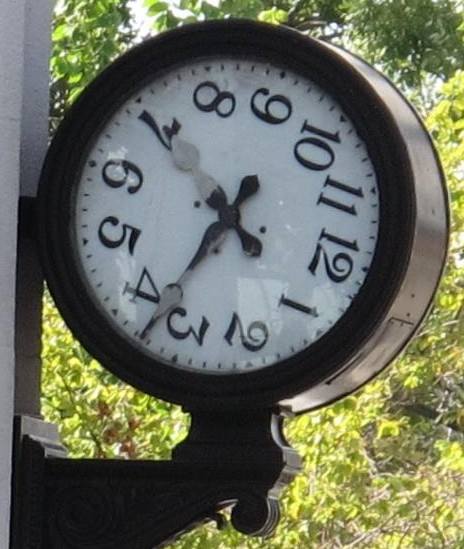In this picture, we see an old-fashioned, ornate clock mounted on a stucco gray building. The large, Victorian-style clock is notable for its unusual orientation: the 12 o'clock position is shifted around to approximately where the 4:30 position should be, creating a tilted appearance. The clock, which is a rich coffee brown with intricate, swooping designs, features black numbers against a white face, each hour individually marked and minute markings around the circumference. The black, slightly worn hands contribute to its vintage aesthetic. In the background, a lush, green tree with visible leaves and branches partially obscures a clear sky, adding a touch of nature to the scene. The entire setup is visually striking due to the clock's substantial size and its peculiarly rotated position.